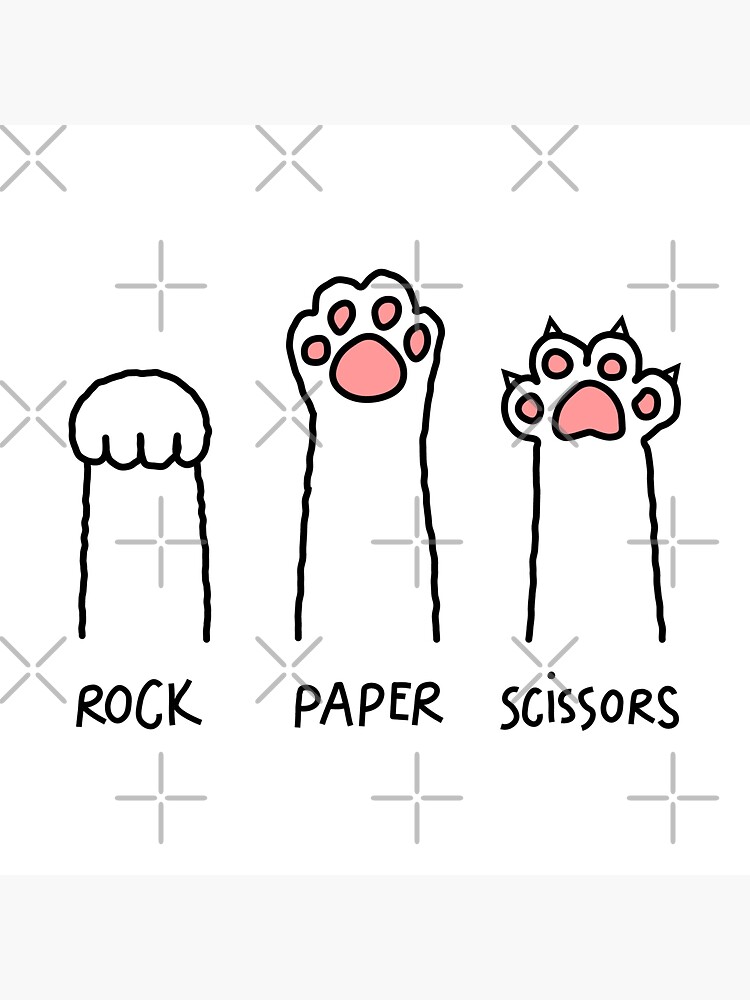The illustrated image presents three different cat paws, each captured in various positions. On the left, a paw is depicted with its pads hidden and is labeled "Rock." The central paw is fully open, showing its pink pads, and is labeled "Paper." The rightmost paw is also open, revealing its pink pads and extended claws, and is labeled "Scissors." The illustrations are rendered in simple black outlines against a white background with pink details on the pads. A light gray watermark featuring a repeating pattern of X's and crosses spans the image, and a light gray bar runs horizontally across the top and bottom edges.